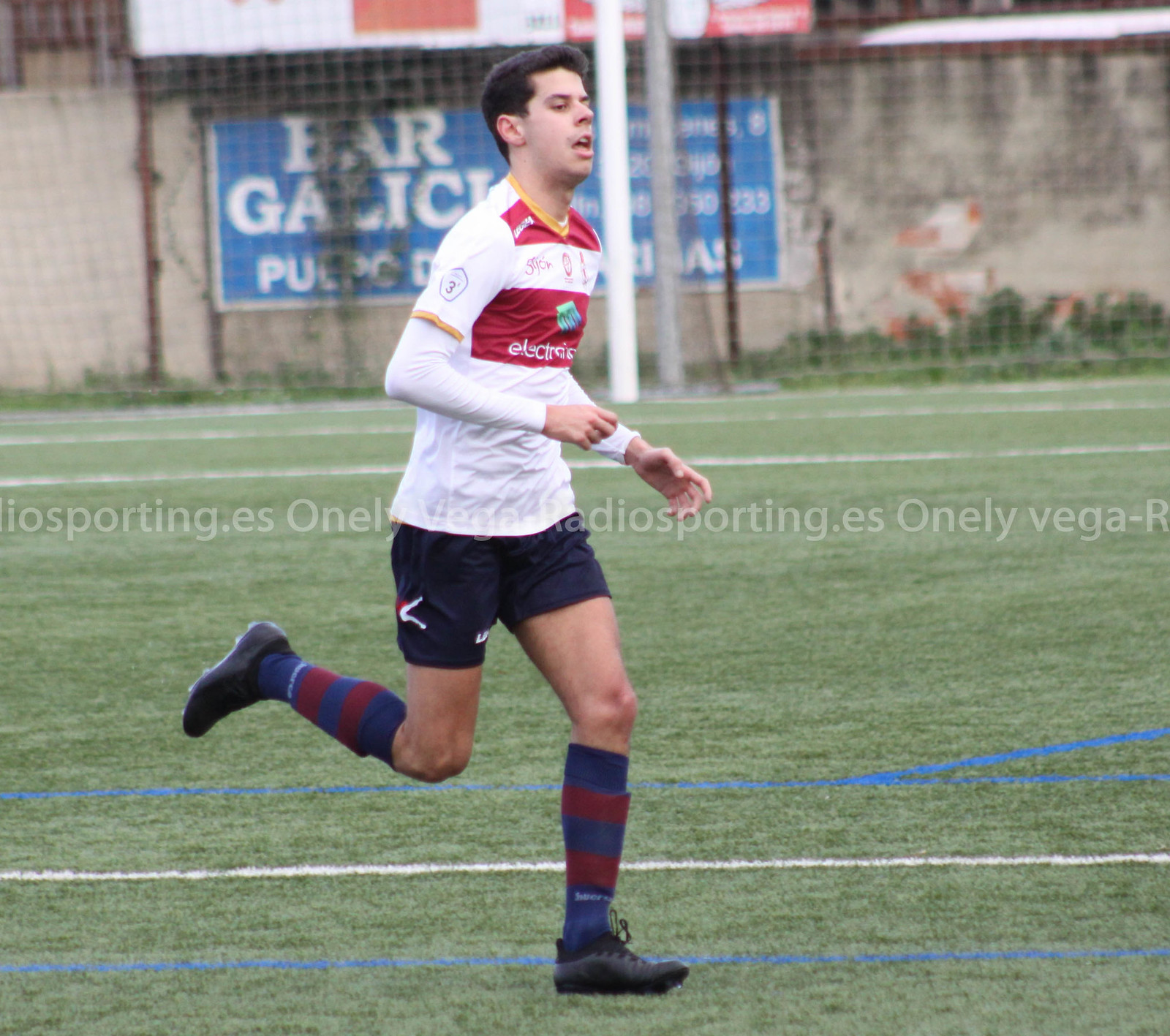The image depicts a male soccer player in mid-run across a green grass field during the daytime. The player has short brown hair and an olive complexion. He is wearing a white and red-striped jersey, which includes a logo or company advertisement on the front, though partially obscured by wrinkles. There is gold trim around the collar and sleeves of the jersey. He is also donning dark blue shorts and knee-high socks that feature dark blue and dark red stripes, along with black cleats.

The field has visible white and blue painted lines and, in the background, a gray, aged concrete wall adorned with dirt and topped with brick. A goal post is faintly visible, along with netting spanning the backdrop. A blue rectangular banner with white text, somewhat obscured by poles and netting, is attached to the fence behind him. Additionally, some text appears on the field that is slightly masked by the player's torso, leaving it partially legible as "onelevega-r" and "iosporting.es." The player appears to be in motion, possibly fatigued with his mouth open, and preparing to kick a soccer ball with one foot lifted and the other planted on the ground.